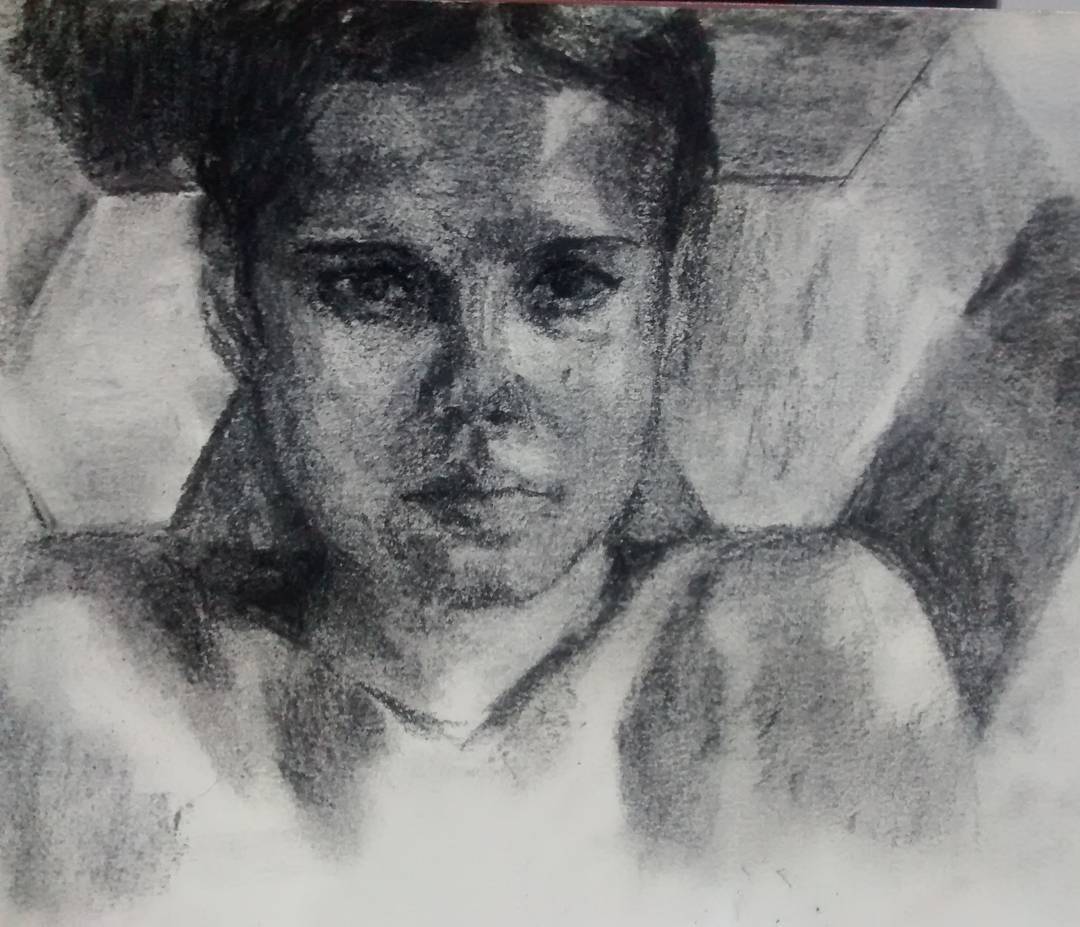A black and white pencil sketch captures a youthful figure, likely female, with prominent facial features centered in the composition. The subject's dark, richly shaded hair frames a face portrayed with meticulous detail. Her eyes, steady and direct, peer out from the page, engaging the viewer with an intense, unwavering gaze. The artist has skillfully rendered her nose and closed lips, adding to the overall clarity and lifelike quality of the drawing. Her shoulders, also visible in the image, appear to be unclothed, though this detail remains subtly ambiguous. The background is left undefined, drawing all attention to her expressive visage and the intricate pencil work that brings it to life.